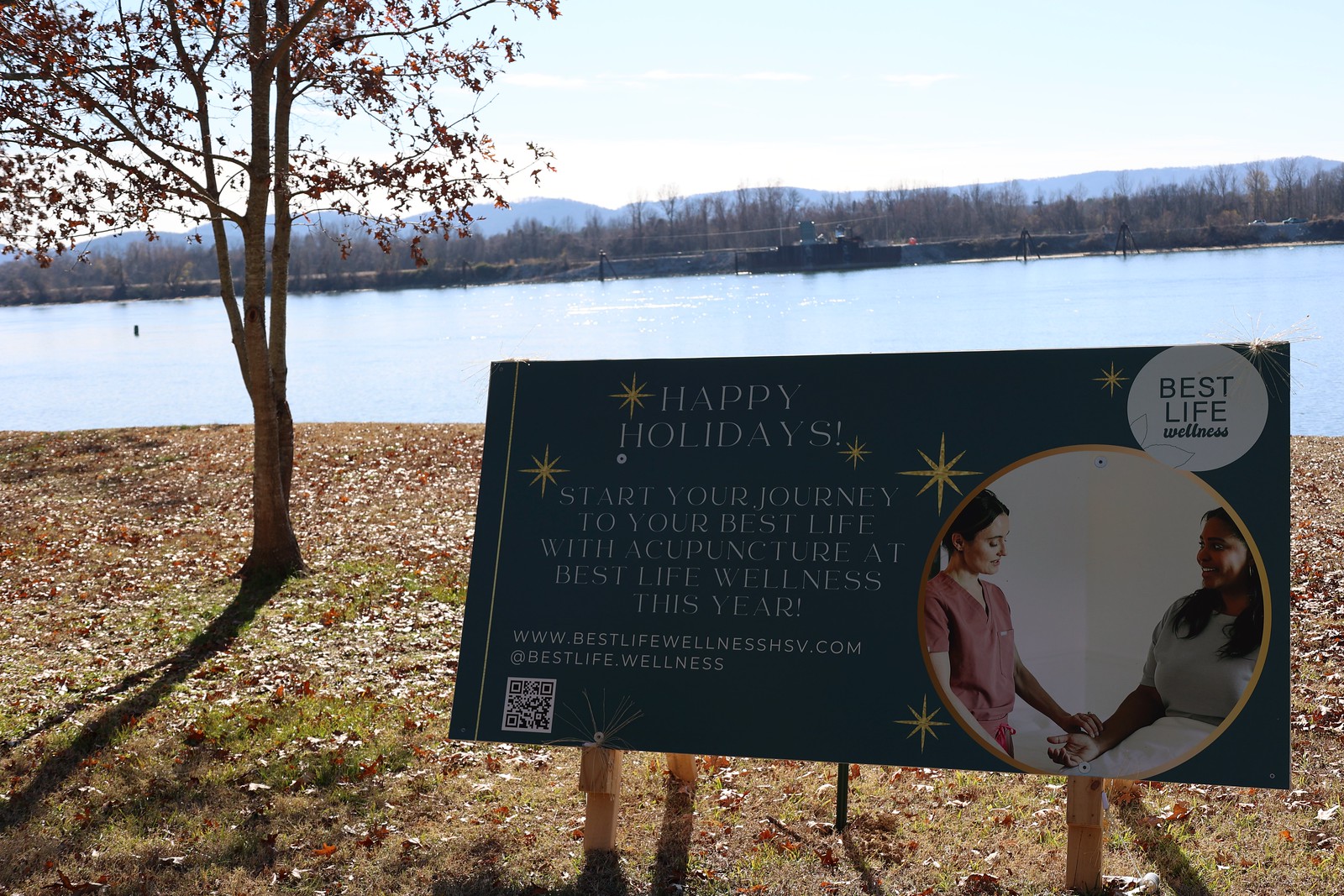In this daylight photograph, a small billboard stands prominently against a serene natural backdrop. The sign is mounted on wooden 2x4 supports and is set in an area with sparse, dead grass and scattered fallen leaves. Behind it is a bare tree, nearly devoid of leaves, with a good-sized pond or small lake stretching out in the background. The horizon reveals a strip of distant mountains, contributing to the picturesque setting. 

The sign itself has a solid navy blue background, adorned with glittery stars that accentuate the festive text. Written in white font on the left side of the board, the message reads: "Happy Holidays! Start your journey to your best life with acupuncture at Best Life Wellness this year," followed by their URL, www.bestlifewellnesshsv.com. A QR code is also located in the bottom left corner. 

Occupying the upper right corner is the Best Life Wellness logo, and below it, a circular photo depicts a nurse, dressed in scrubs, gently holding the hand of a smiling patient, perhaps taking their heart rate. The scene harmoniously blends the warmth of holiday wishes with the promise of wellness and care, inviting viewers to embark on a journey to better health.